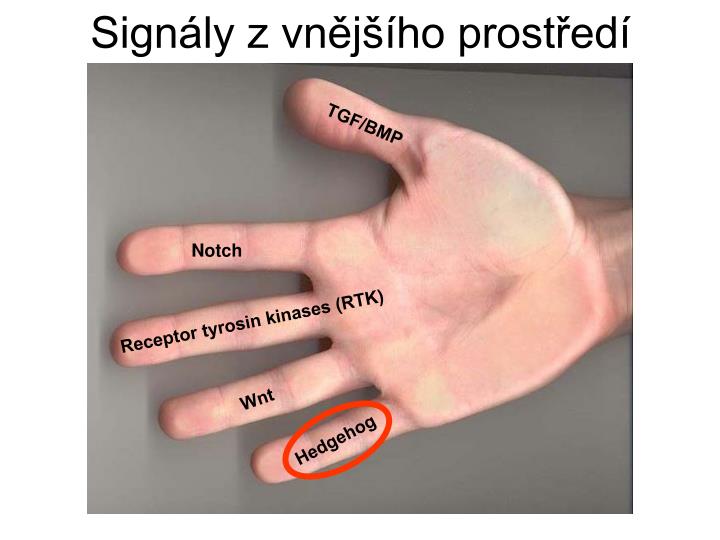The image features a detailed diagram of a right hand with outstretched fingers, positioned palm-up against a gray background. At the top of the image, there is a title in black font that reads "Signali zi venjtijo prostreti," suggesting the image is in a non-English language. Each finger on the hand is labeled with specific scientific terms: the thumb reads "TGF/BMP," the index finger is labeled "Notch" (with a capital 'N'), the middle finger has "Receptor Tyrosine Kinases (RTK)" written on it, the ring finger is marked "WNT," and the pinky finger is labeled "Hedgehog," emphasized by an orange oval around the word. The hand and its annotations are set against a muted gray background, which varies in shade, and the overall composition might be used for educational purposes, such as in a medical or biological context.